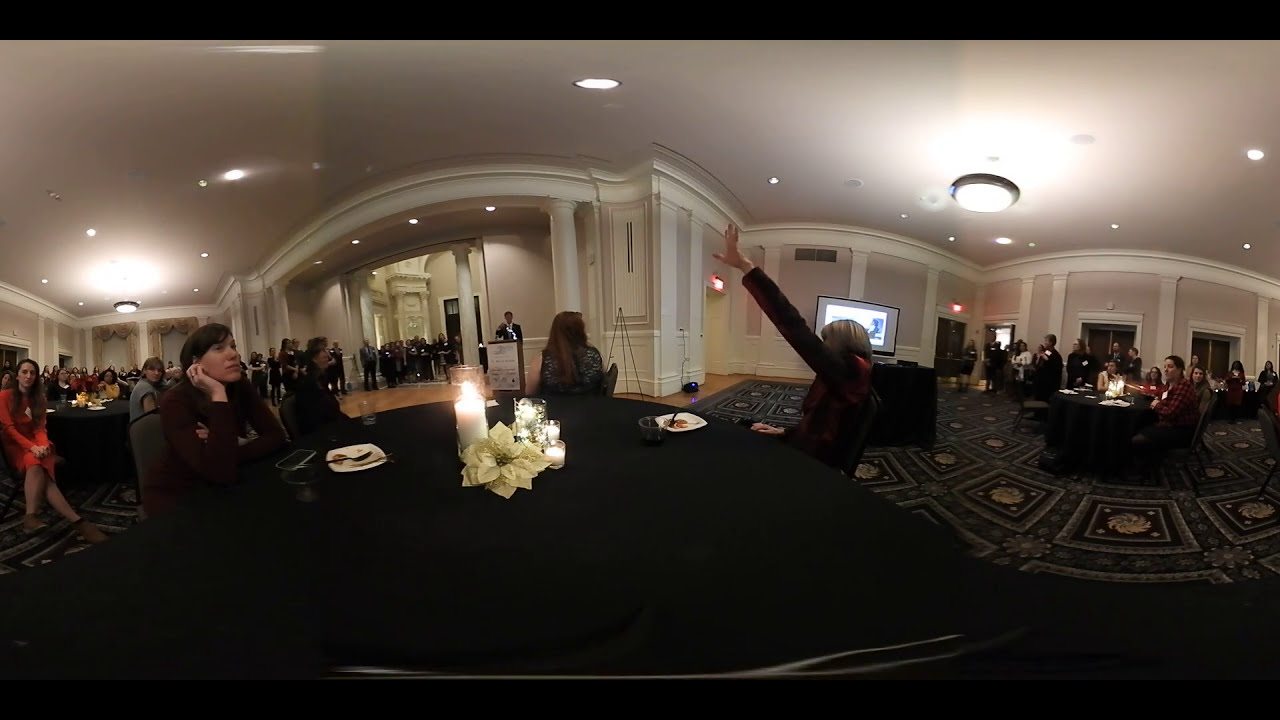The image depicts a bustling conference or event taking place in a uniquely designed room with rounded, bubbly archways and white, cream-colored walls and ceilings, adorned with columned architecture. The panoramic shot captures numerous black tables scattered throughout the room, each adorned with small white plates, lit glass candles, and arrangements featuring a tall white candle and a large white flower. At the center is a prominent black round table where three women sit; one in a dark red dress with her back turned, one in a black outfit with her left hand raised, and another simply gazing around. Surrounding them, the room is filled with smartly dressed attendees, either seated or standing. The carpet on the ground is a complex design featuring dark squares and circular decorations. On the center right, a presentation screen and projector are visible, and on the right side of the room, there's a wooden podium with a person in a black suit standing behind it. The scene is lively, with clusters of people engaging near doorways and entryways equipped with lighting.